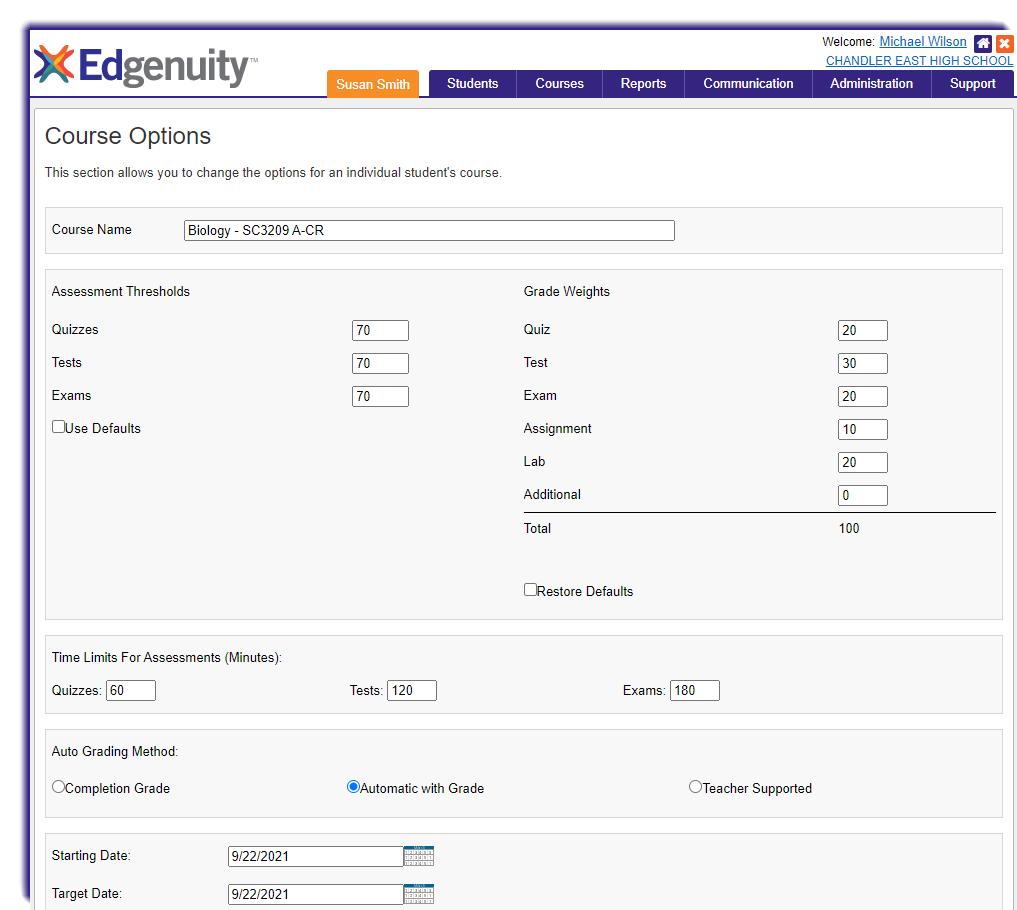The image depicts a class registration interface for a school using the Edgenuity platform. On the left side, there is a green "X" mark contrasted by an orange "X" on the right side, with the word "Edgenuity" prominently displayed. 

In the main section, there are various colored boxes, including an orange box labeled "Susan Smith" and several adjacent purple boxes delineated as "Students," "Courses," "Reports," "Communication," "Administration," and "Support."

At the top of the interface, a welcome message reads, "Welcome, Michael Wilson, Chandler East High School," accompanied by a small home icon and an orange "X" in the top right corner. Below this, a section entitled "Course Options" is visible, which allows adjustments to individual student course settings. 

The course name selected is "Biology-SE2309A-CR." For assessment thresholds, the interface lists "Quizzes," "Tests," and "Exams" with input boxes set at "70" for each. A checkbox labeled "Use Defaults" is present but not checked. 

Under "Grade Weights," the details include:
- Quiz: 20
- Test: 30
- Exam: 20
- Assignment: 10
- Lab: 20
- Additional: 0
- Total: 100

There is a checkbox for "Restore Defaults," which is also unchecked. All these values are contained within editable text boxes. 

The "Time Limits for Assessments" section specifies:
- Minutes for Quizzes: 60
- Tests: 120
- Exams: 180 

The "Auto Grading Method" offers three options: "Completion Grade," "Automatic with Grade," and "Teacher Supported," with "Automatic with Grade" being selected, marked by a blue circle.

Finally, there are fields for the "Starting Date" and "Target Date" both set to "9-22-21," with calendar widgets available for selection.